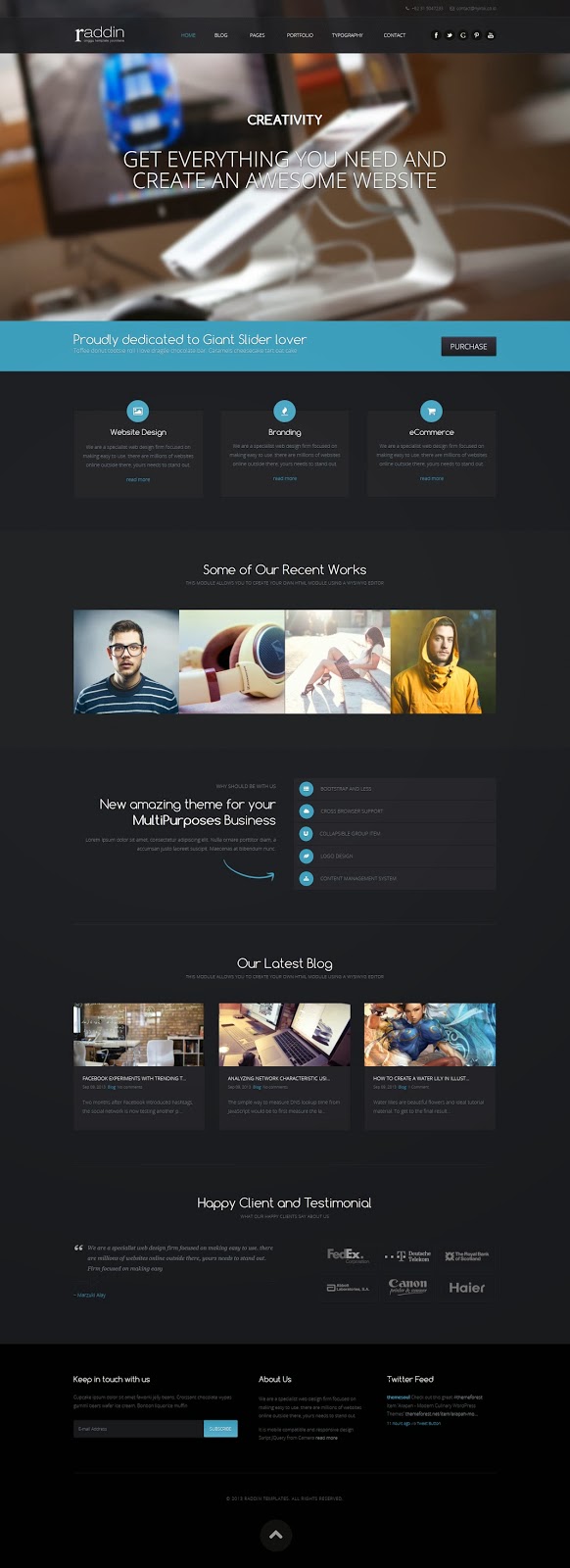**Website Overview Screenshot Caption:**

The image captures a detailed screenshot of a website named "RADIN". In the upper left corner, the website's name "RADIN" is displayed prominently in white text. To the right, a navigation bar includes links to "Home", "Blog", "Pages", "Portfolio", "Typography", and "Contact". Further right, there is a section with circular social media icons representing Facebook (F), Twitter (bird), Google+ (G), Pinterest (P), and YouTube.

Beneath the header, there is a picture taken from an oblique angle of a home office setup, featuring an Apple display monitor and a MacBook on a stand. The image is slightly out of focus, showing a black mouse and keyboard on the desk. Overlaid on this image is the word "Creativity" in white text, followed by the tagline "Get everything you need to create an awesome website."

The next section features a blue background with white text reading "Proudly dedicated to giant slider lovers," and a black "Purchase" button on the right-hand side. Following this, there are three units (or "divs" in web development terms) labeled "Website Design," "Branding," and "e-Commerce," each with a corresponding blue circle icon: a picture icon, an unidentified icon, and a shopping cart icon, respectively. These units are presented on dark gray squares with white text.

Further down, a section titled "Some of Our Recent Works" is shown, with four horizontally aligned images. Below, a new section titled "New Amazing Theme for Your Multi-Purpose Businesses" appears in white text, accompanied by an arrow that points to vertically listed sections. 

Subsequently, there is a section labeled "Our Latest Blog," displaying three blog post previews with images at the top and details such as title, date, author, and snippets of content at the bottom.

The following section contains testimonials under "Happy Client and Testimonials," featuring logos of partner companies and client quotes. 

At the bottom of the webpage, the footer includes an input field for subscribing via email, an "About Us" section, and a Twitter feed. The footer concludes with copyright information and an arrow for scrolling back to the top of the page.